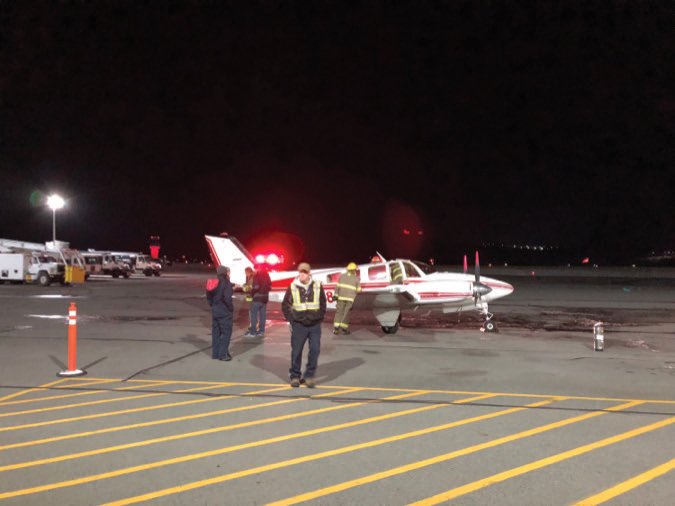In the middle of a pitch-black night at an airport landing strip, a small white airplane with red stripes and dual front propellers catches the intense beams of spotlights. The plane, possibly designed for one or two passengers, is surrounded by four or five individuals, including at least two firefighters inspecting the interior, suggesting a potential issue upon landing. Nearby, a man in a bright construction vest and brown hat looks away, while other onlookers, dressed in dark clothing, converse among themselves. To the left, several gray utility trucks, some equipped with ladders, stand illuminated by the spotlights. The scene is punctuated with red lights, yellow angled stripes painted on the concrete, and an orange safety cone, adding to the chaos of the scene.